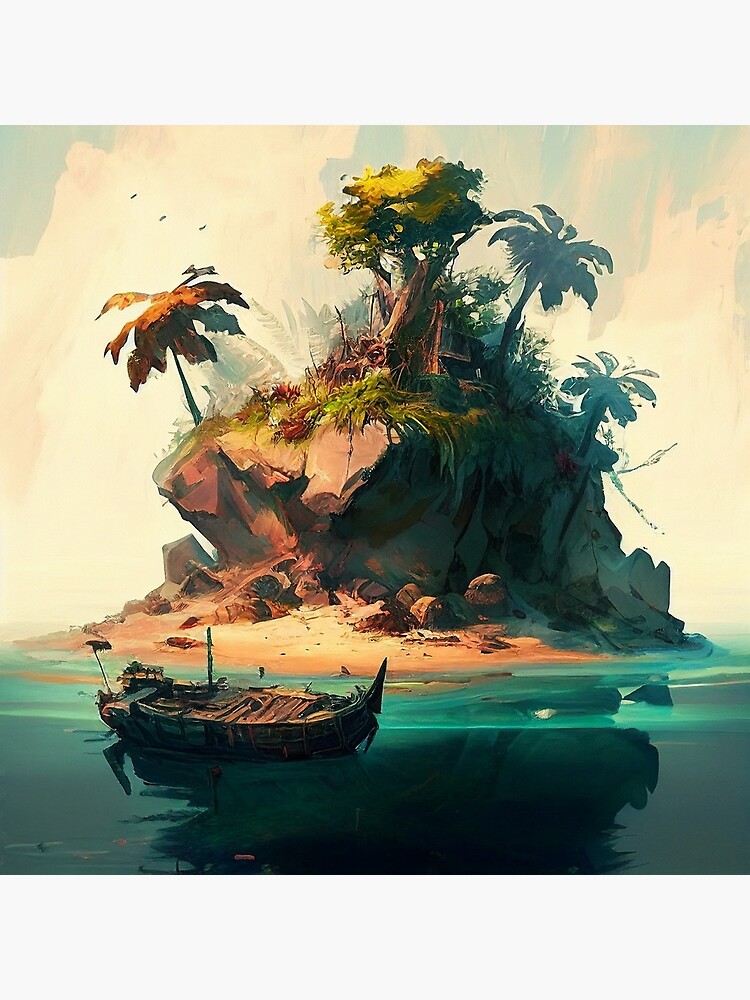In this evocative painting, a dilapidated wooden boat, tilted to the left with broken wood inside, rests at the base of a minuscule, round island. The island is scarcely larger than the boat itself, a patch of rusty brown and tan sand dominated by a massive rocky mound. This central rocky structure, which appears fragmented as if torn from a larger landmass, rises significantly above the island with a height ranging from 20 to 40 feet. The rocky surface is adorned with patches of green grass and various trees—some resembling palm trees with rusty brown trunks and faded green fronds, and others akin to traditional deciduous trees. 

A vague wooden structure, partially obscured by foliage, crowns the top of the island. Jagged rocks jut out from the turquoise and multicolored blue water that shifts to sea green and pea green hues near the shore. The shoreline itself is strewn with boulders, adding to the rugged, desolate scene. Overhead, the sky is a hazy white with hints of light green in the corners, and a few birds can be seen flying in the distance. The entire scene is framed with a broad white border at the top and bottom, enhancing the image’s artistic composition.